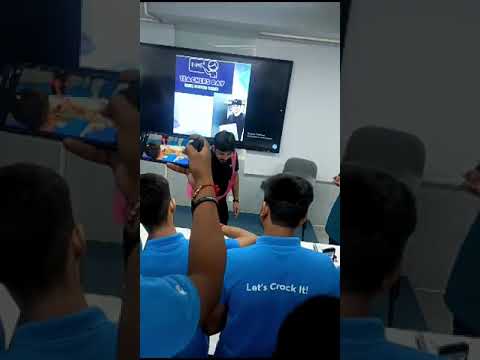The image is a vertical cell phone photograph depicting an educational class in progress. The main focus is on several audience members wearing matching blue polo shirts, one of which has the slogan "Let's crock it!" on the back. The scene is viewed from the perspective of one of these attendees, looking towards the instructor at the front of the room. The instructor, identifiable by a pink reflective jacket worn over a black shirt, stands before a gray drywall wall. This wall features a large flat-screen television displaying an infographic, most likely related to the training taking place. The camera’s vantage point shows a few empty chairs scattered among the audience members, some of whom appear to be capturing the session on their phones. The image is bordered on both sides by a zoomed-in and faded version of the same scene, giving it a triptych-like appearance.